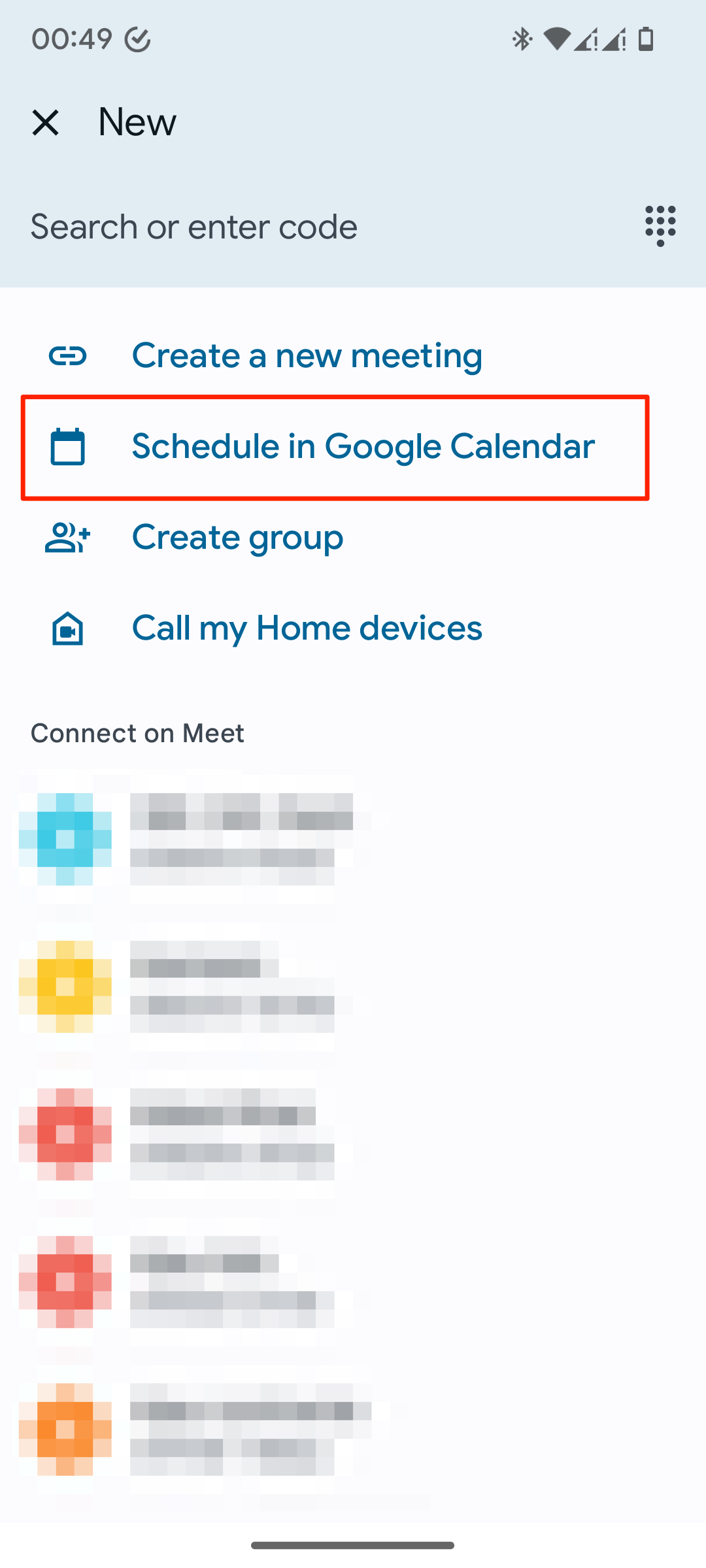This screenshot captures the interface of a mobile phone screen with various displayed elements. In the top-left corner, a small timer with a gray background and black text reads "00:49," accompanied by a circled check mark. Meanwhile, the top-right corner features several phone status symbols: a Bluetooth icon, a nearly-drained battery icon, a strong Wi-Fi connection indicator, and an internet signal icon marked with an exclamation point indicating an issue.

Below these indicators is a black "X" with the word "New" beside it. Directly beneath, there's a search bar prompting "Search or enter code," next to a 3x3 grid icon representing additional options. Following this, in blue text, are options to "Create new meeting," and underneath, a red-bordered option to "Schedule in Google Calendar." Further down the interface, options to "Create group" and "Call my home devices" are listed, followed by a smaller black text link that reads "Connect on Meet." At the bottom, there are five blurred-out pictures, presumably representing users or contacts.